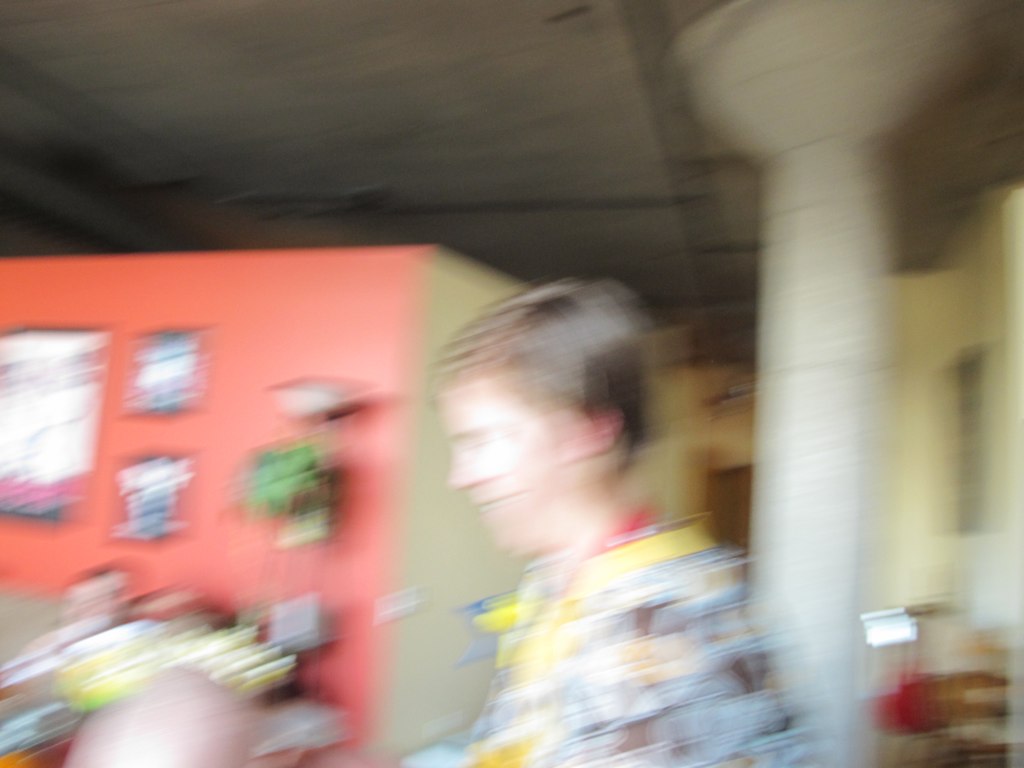A slightly out-of-focus photograph captures a joyful individual situated in the lower central-left portion of the image. The person, facing towards the left, is caught in a smile, their brown hair neatly trimmed just above the ears. They don a jacket with hues of yellow and muted yellow, accented possibly with touches of white and blue. Directly behind this individual stands a white pillar that stretches up to meet a black ceiling. To the left and behind, a cube-shaped wall serves as a backdrop, with one side painted in a rose color and the other in a yellow tone. The wall is adorned with various hanging objects, adding to the scene's visual interest. Additionally, the partial presence of another individual can be detected in front of the main subject, identified only by a bald head and an ear.